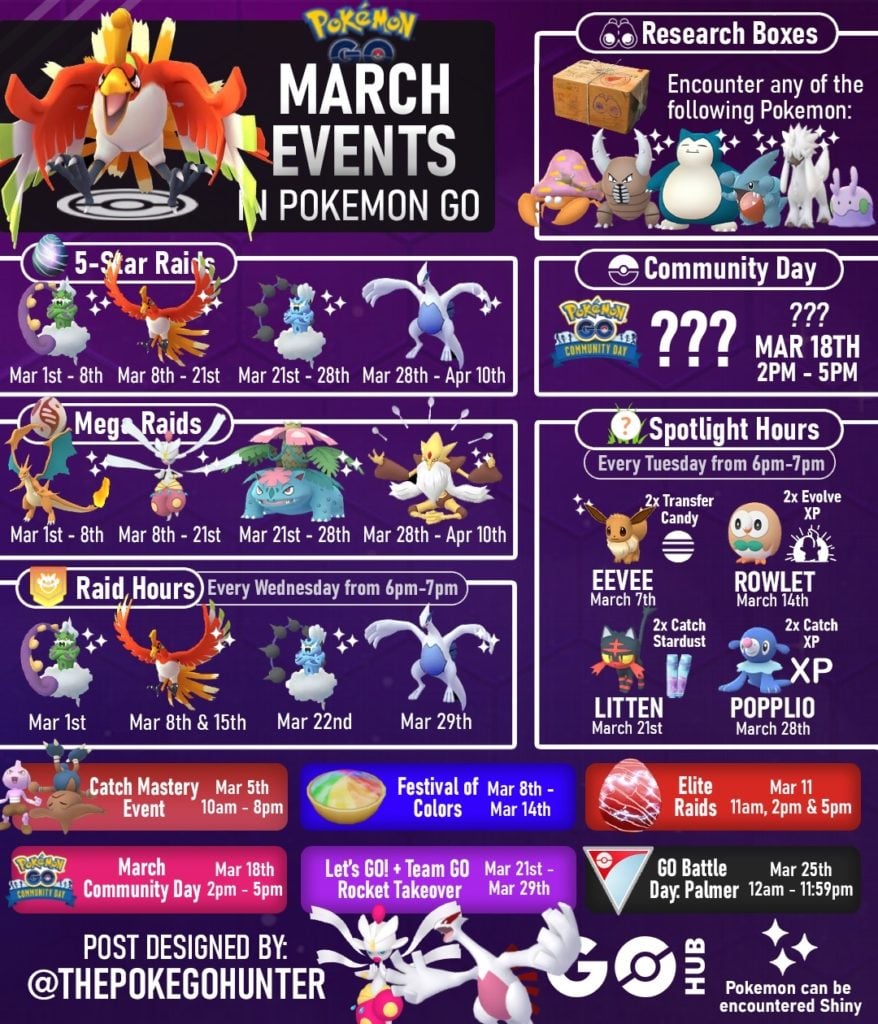**Detailed Caption for the Image:**

The image prominently features the "Pokémon GO" logo at the top, rendered in yellow with a blue outline that gives it a three-dimensional effect. Below the logo, "GO" is written in navy and outlined in gray. In large white letters, the words "March Events" are displayed, highlighting the content of the image, which is focused on "Pokémon GO." 

At the center of the image, a majestic bird with bright orange wings is showcased, symbolizing the main event. Below the bird, the text "Five Star Raids" is displayed. Key raid periods are listed sequentially:
- March 1st to the 8th
- March 8th to the 21st
- March 21st to the 28th
- March 28th to April 10th

Each date range is accompanied by small bird icons that represent the Pokémon available for the raids.

Next, the heading "Mega Raids" is featured along with corresponding date ranges:
- March 1st to the 8th
- March 8th to the 21st
- March 21st to the 28th
- March 28th to April 10th

Similarly, cartoon-like characters symbolizing featured Pokémon are displayed above each date range.

Following that, "Raid Hours" are announced, specifying every Wednesday from 6 PM to 7 PM:
- March 1st
- March 8th
- March 15th
- March 22nd
- March 29th

Again, these are accented with small cartoon bird characters.

The image also lists various events:
- "Catch Mystery Event" on March 5th from 10 AM to 8 PM
- "March Community Day" on March 18th from 2 PM to 5 PM

In the middle section, a blue banner reads "Festival of Colors" from March 8th to March 14th. Below it, a purple banner declares, "Let's Go, Rocket Takeoff, Team GO" from March 21st to 29th. 

On the right side of the image, a red banner announces "Elite Raids" on March 11th at 11 AM, 2 PM, and 5 PM. Below, "Go Battle Day Palmer" runs on March 25th from 12 AM to 11:59 PM. 

At the top right, there's information about "Research Boxes," indicating players can "Encounter Any of the Following Pokémon," accompanied by various Pokémon images.

Further down, another mention of "Community Day" emphasizes March 18th from 2 PM to 5 PM with three white question marks.

"Spotlight Hours" are detailed, scheduled every Tuesday from 6 PM to 7 PM, offering bonus features like double Transfer Candy and double Evolve XP. Specific dates and Pokémon are listed:
- Eevee on March 7th
- Rowlet on March 14th
- Litten on March 21st
- Popplio on March 28th

Finally, at the bottom, the caption credits "Post Design by @PokeGoHunter," with additional cartoon-like characters and a note that says "Pokémon can be encountered shiny."

This comprehensive list of events and their corresponding visuals offers players a detailed schedule for March's activities in "Pokémon GO."